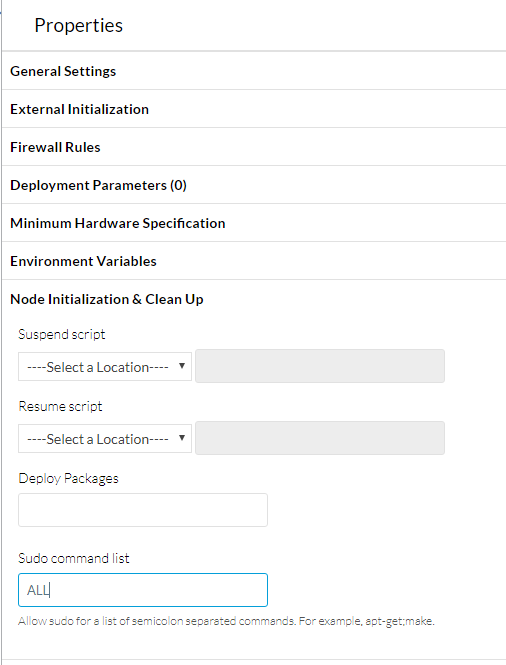The image is a screenshot of a settings page with a white background and black text, divided by light gray horizontal lines. A light gray vertical line runs down the left side of the page. The header at the top of the page reads "Properties". The settings are categorized and listed in sequence from top to bottom: General Settings, External Initialization, Firewall Rules, Deployment Parameters, Minimum Hardware Specification, Environment Variables, Node Initialization, and Cleanup. The Cleanup section is currently selected, revealing multiple input fields including drop-down menus and text boxes. The visible options under Cleanup are: Suspend Script, Resume Script, and Deploy Packages. Beneath Deploy Packages is a text field labeled "Sudo Command List", in which the word "all" has been entered.